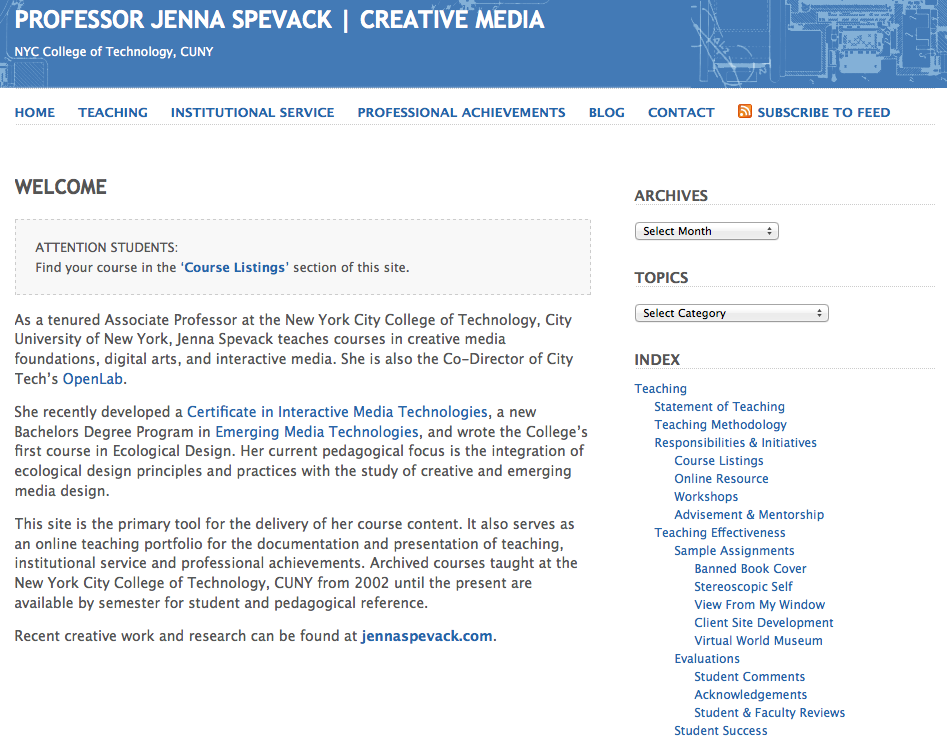The screenshot depicts a webpage that serves as the online professional profile of Professor Jenna Spivak, who specializes in Creative Media at the New York City College of Technology, part of the City University of New York (CUNY) system. The webpage features a clean, primarily white background with a medium blue border at the top. The blue border includes a subtle, stylish graphic reminiscent of computer chip designs on the right side. 

In this blue header, the text reads "Professor Jenna Spivak, Creative Media," followed by "NYC College of Technology, CUNY" in white font. Beneath this, a navigation bar presents clickable options: Home, Teaching, Institutional Service, Professional Achievements, Blog, Contact, and Subscribe to Feed.

The main section of the page welcomes visitors with a "Welcome" message in black or gray print. Below, it addresses students, instructing them to find their courses in the "Course Listing Selection" section. 

In an introductory message, Professor Spivak, a Tenured Associate Professor, outlines her role and contributions at the college. She teaches Creative Media, Foundations, Digital Art, and Interactive Media courses. Notably, she serves as co-director of City Tech's Open Lab and has spearheaded several academic initiatives. These include the development of a certificate in Interactive Media Technologies, a bachelor's degree program in Emerging Media Technologies (which is highlighted in a lighter blue text), and the creation of the college's first course in Ecological Design.

On the right side of the page, a column features additional selectable options, such as Archives (with a dropdown menu for selecting the month), Topics (with a dropdown for categories), and an Index. Under the Index, subcategories include Teaching, Statements of Teaching, Teaching Methodologies, Responsibilities, and Initiatives.

This detailed profile showcases Professor Spivak's extensive academic contributions and is likely her professional webpage within the college's domain, highlighting her teaching, research, and program development efforts.